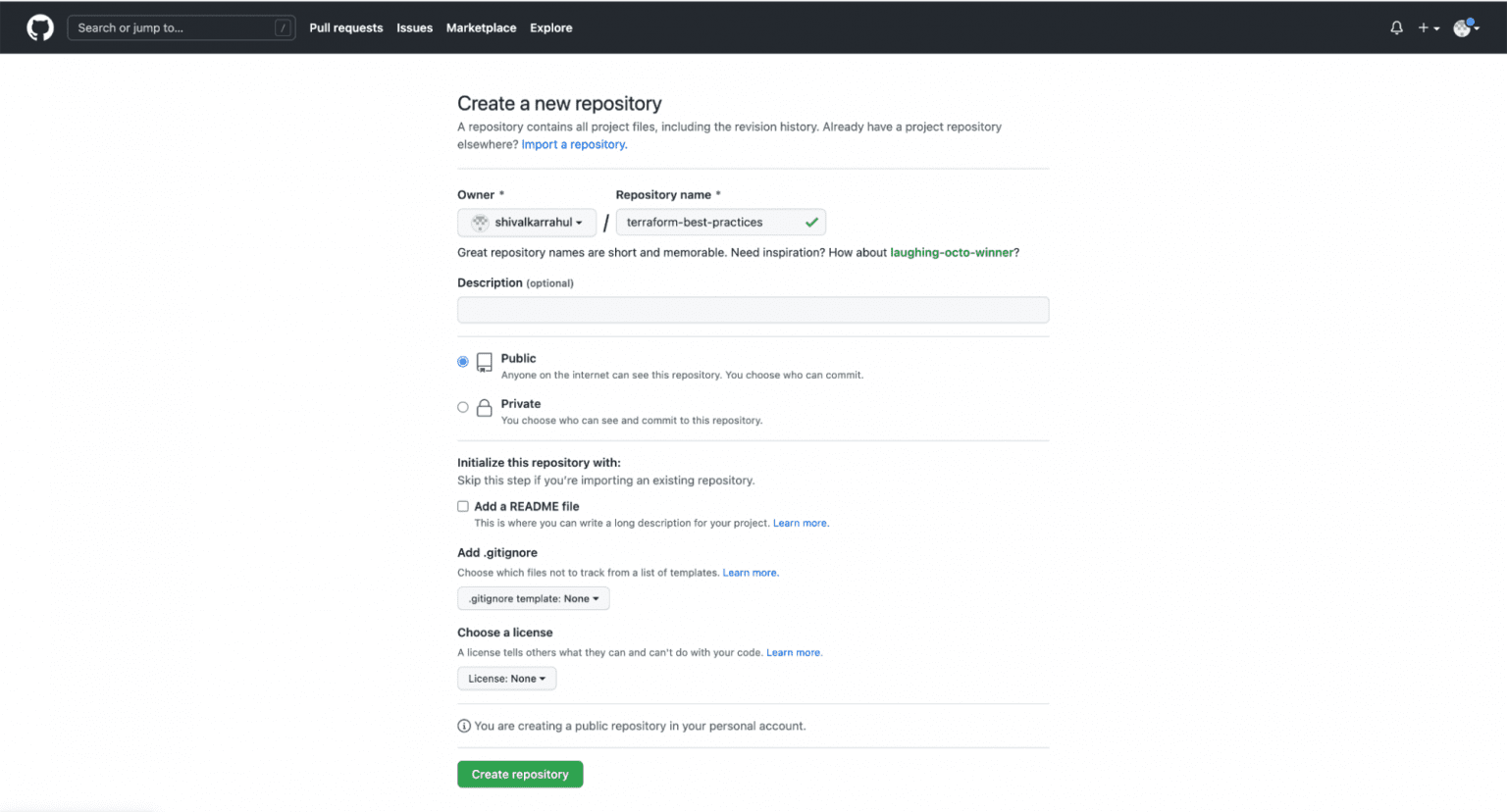The left-hand side of the image features a circular logo with a white background, displaying a silhouette of a cat with its right arm extended. To the right of the logo, there is a search bar labeled "Search or jump to." Continuing rightward across the top menu, the following options are visible: "Pull requests," "Issues," "Marketplace," and "Explore." 

In the upper right-hand corner, the interface includes several icons: a bell notification symbol, a plus sign with a drop-down arrow, and a circular profile picture indicating the user’s login status. 

Below the top menu, the main screen content is centered around the title "Create a New Repository." Under this title, there are fields for the owner's name and the repository's name. At the bottom of this section, a "Create Repository" button is prominently displayed. The overall layout is clean and organized, providing a clear pathway for users to create a new repository on the platform.